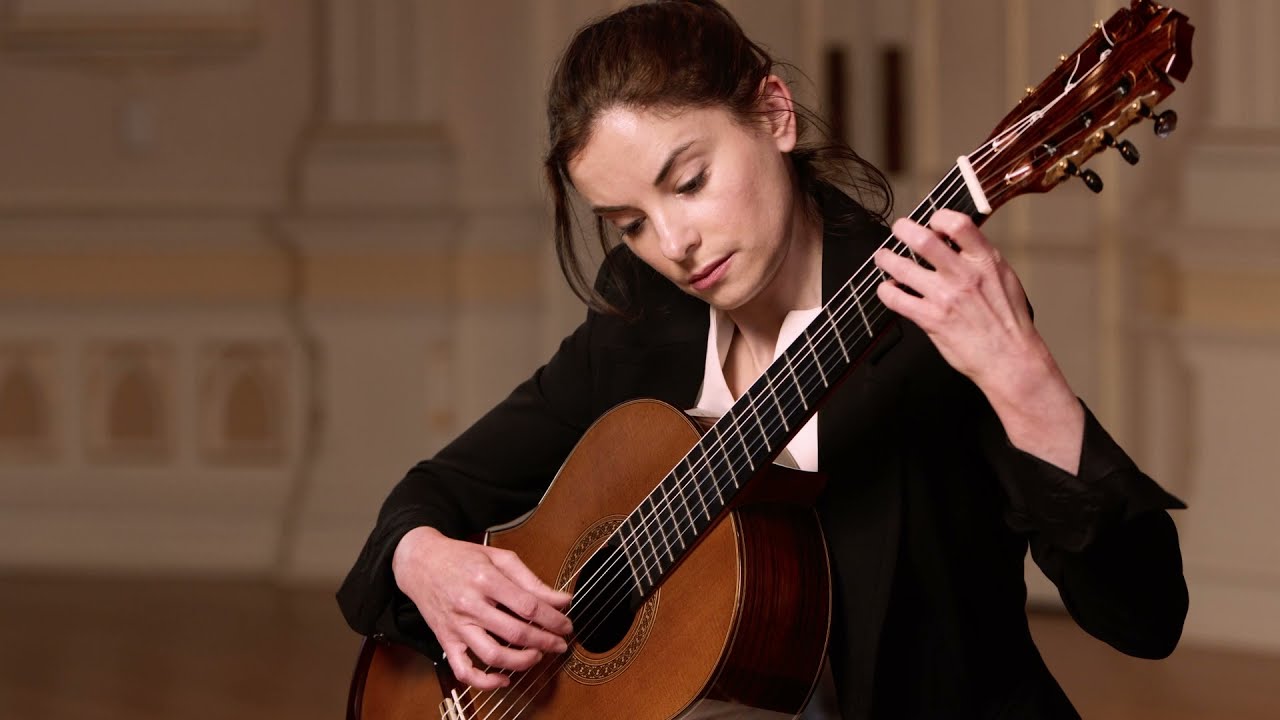This is a detailed image of a white woman, shown close up, deeply engrossed in playing a large, dark brown guitar. She is a brunette, likely with her hair pulled back into a ponytail, though some strands hang down to the right. She wears a black suit jacket over a white blouse, with the open neckline adding a subtle contrast. Her gaze is focused downward, intently concentrating on her music. In her right hand, she strums the guitar, while her left hand deftly maneuvers the frets, with four fingers visibly pressing the strings. The guitar itself is shiny on its sides and top, and its head features numerous tuning points. The background is muted and blurry, highlighting the elegant architecture of what appears to be a fancy performance room with white and yellow accents on the walls. This setting suggests she might be performing a classical or flamenco piece, possibly during a recital or an audition, her expression conveying a sense of contemplation and dedication to her craft.